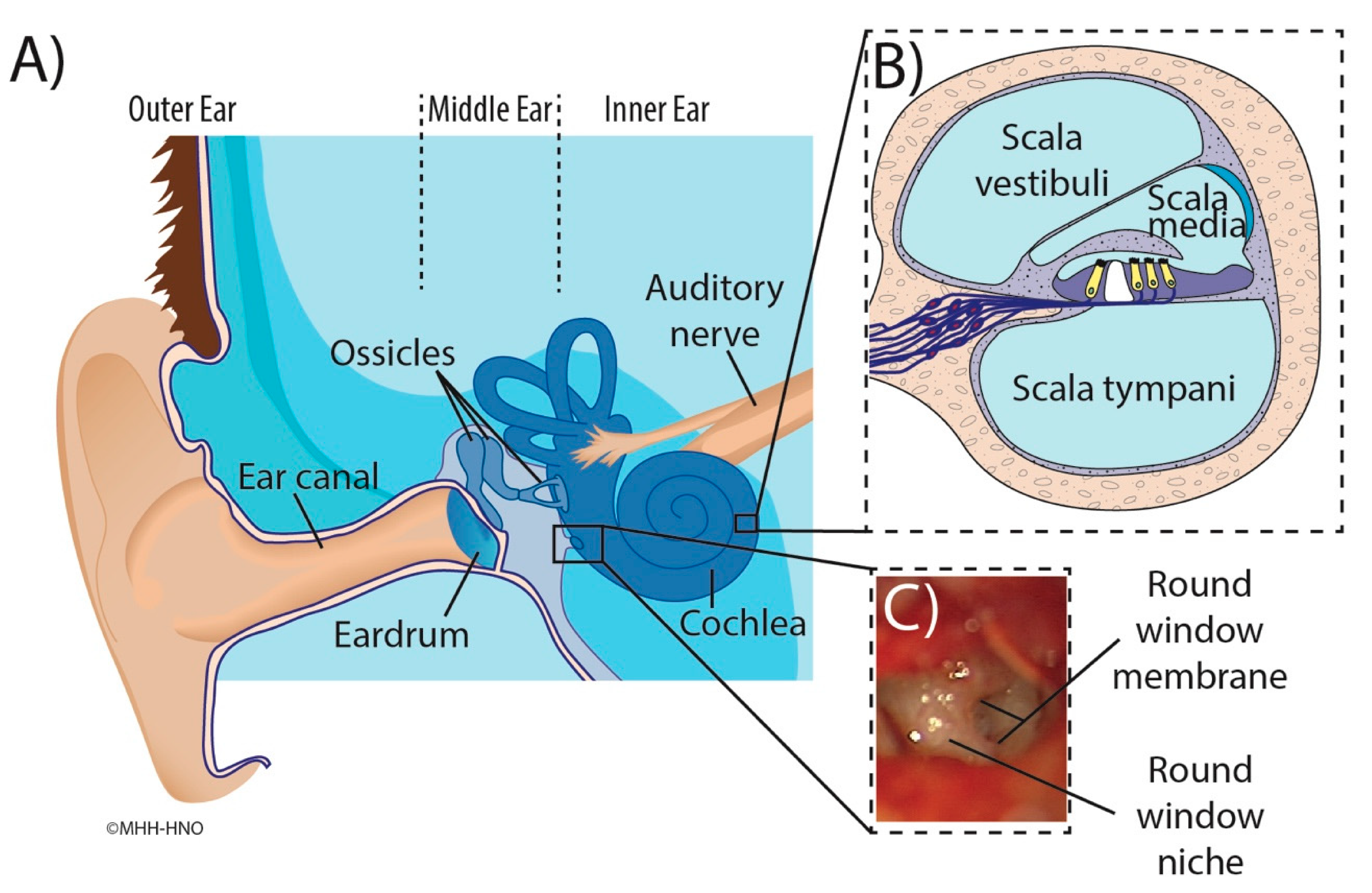This is an image divided into three sections, showcasing a detailed diagram of the ear, combining colored drawings and a photograph. In the upper left corner, it begins with a labeled section (A) set against a white background, featuring a cartoon-like depiction of the ear's anatomy. The outer ear is illustrated in a tan hue, transitioning to a blue-colored middle ear and inner ear. Key parts of the ear are annotated, including the ear canal, eardrum, ossicles, cochlea, and auditory nerve, each labeled with black text. 

To the right, there's another section labeled (B) with a dashed border, illustrating the internal structures of the cochlea. This part of the diagram notably resembles an oval, with colorful segments and labels for scala vestibuli, scala media, and scala tympani, depicted in shades of pink, blue, yellow, purple, and white.

The final section below is marked as (C) in a rectangle with a dotted border, showcasing an actual photograph rather than a drawing. It presents a realistic image of the round window membrane and round window niche, with distinct red and brown hues. This section emphasizes the real-life appearance of these intricate ear structures. The overall diagram uses a color palette of black, white, gray, peach, pink, blue, purple, yellow, red, and brown to clearly differentiate and label each part.